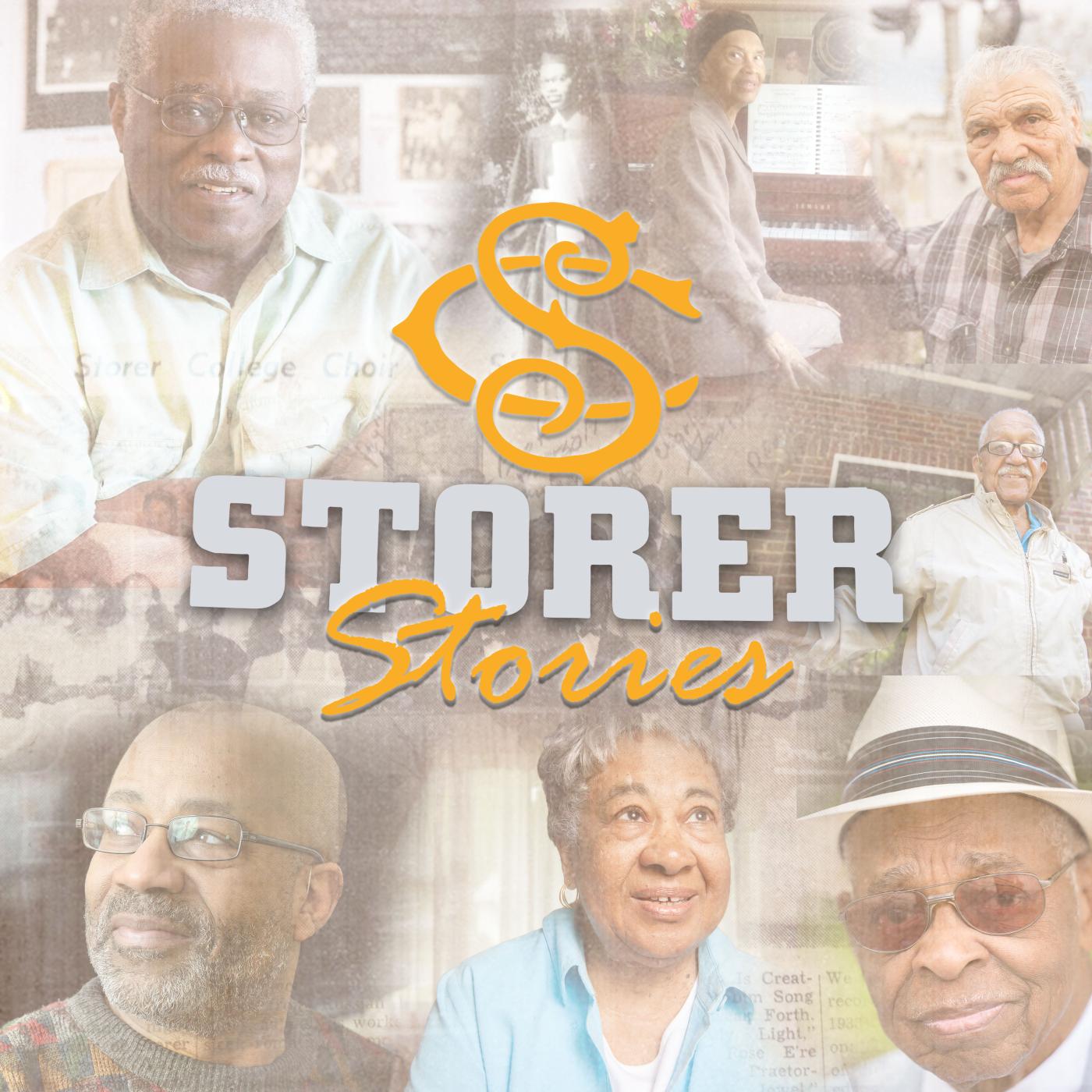The image is a slightly vertical rectangular collage featuring photographs of approximately eight older and elderly individuals, all dressed in various outfits including shirts, t-shirts, and one man in the bottom right corner wearing a hat and glasses. The overall background is somewhat blurred, creating a faded, hazy effect on the photos of the people, emphasizing their smiles and the suggestion that they are sharing personal life stories. 

Centrally placed in the image is text that stands out sharply against the blurry background: a large, orangish 'SC' logo is present just above the center, with 'Tora' written in grey immediately beneath it, and 'Stories' in yellow below that. The top left of the collage features a large photo of a man, and to the right of that sequence are images of two women, one of whom is at a piano, followed by another man. The middle area beneath the 'SC' logo, although obscured, appears to have another image, flanked by photos of a man. Along the bottom are three more images: a man on the left, a woman in the middle, and a man on the right, with an additional image of a group of people located between the leftmost man and the woman. The letters in the middle, 'Tora Stories,' are crisp and distinct, contrasting with the softer, nostalgic tone set by the background collage of faces.